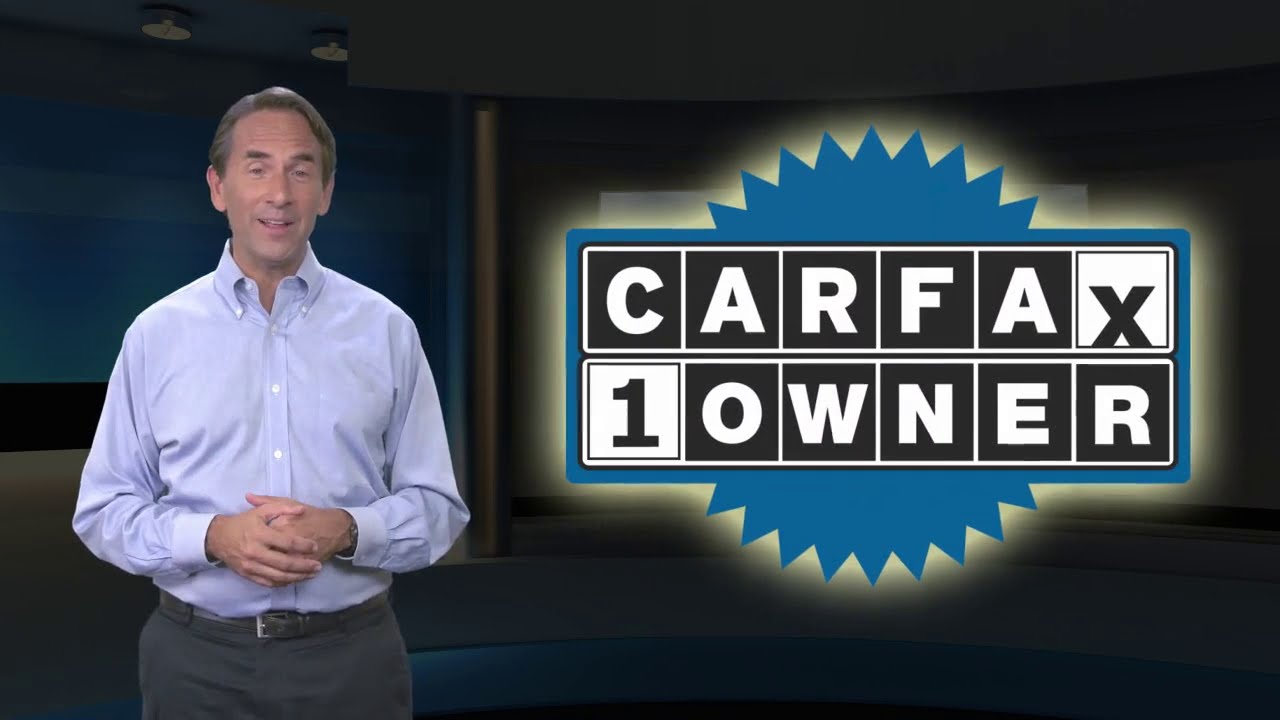The image showcases a Carfax advertisement, featuring a middle-aged man with brownish-gray hair standing to the left. He is wearing a light blue collared, long-sleeved shirt tucked into gray dress pants with a belt, complemented by a watch on his wrist. The man, who appears to be around his 50s, is smiling at the camera with his arms crossed, presenting a poised and professional demeanor. Behind him is a backdrop resembling a green screen, creating a 3D effect with blue and black tones and synthetic lighting.

To the right of the man, a prominent Carfax logo reads "Carfax One Owner," accompanied by a blue ribbon or seal. This well-recognized logo sits in front of a glowing light on the dark background, adding a striking visual element to the composition. The setting appears to be an indoor studio, suggesting that the scene is part of an advertisement presentation for Carfax.